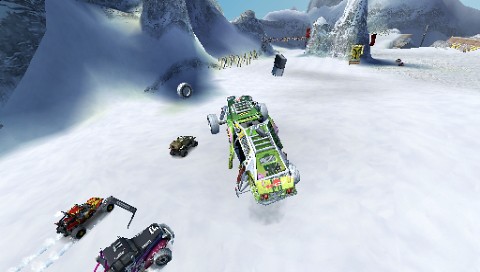This image is a screenshot from a video game, depicting an exhilarating race in a pixelated and slightly dated-looking snowy mountain landscape. In the foreground, a diverse array of vehicles tackle a snowy path laden with obstacles and stone formations of varying shades of gray. Dominating the scene is a larger green vehicle, its vibrant neon and dark green hues reminiscent of a Mountain Dew bottle, which grabs the viewer's attention as it flips dramatically through the air. This vehicle has silvery tires and is flanked by smaller ATVs and dune buggies with distinctive features: a red and yellow car, a mostly black one with magenta sides, and a black and white one. Supporting details include an army-style truck with a loose tire and debris trailing in its wake. To the left, three ATVs race ahead, while in the background, a mix of flags, signs around a large rock, and a snow-covered clearing complete the action-packed scene.